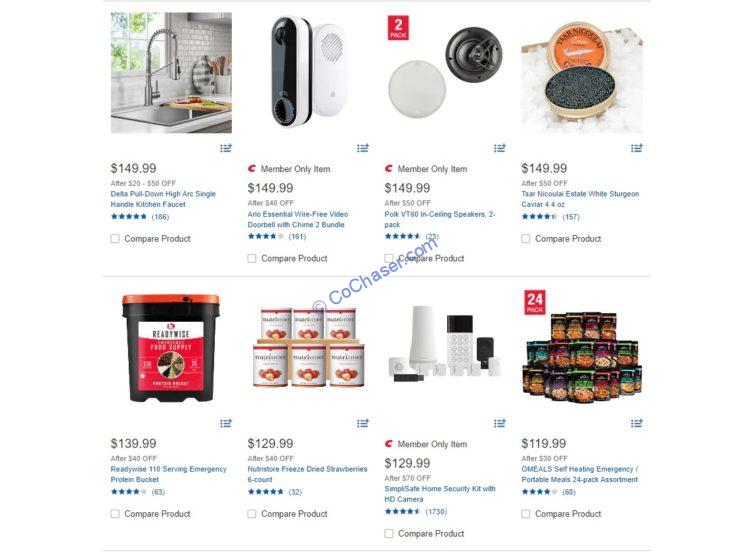**Detailed Caption:**

This web page belongs to Cochaser.com, a website dedicated to selling a diverse range of consumer goods. The page prominently features eight items, organized neatly in two rows of four. Each item is represented by a clear image, catering to various shopping needs.

In the top-left corner, there's a Delta Pure Down Height kitchen sink priced at $149.99, complete with an image showcasing the elegant Delta faucet. To its right, a Members Only item, the Arlo video doorbell, is displayed with a corresponding picture, adding a touch of modern security to the selection.

The third item on the top row is another Members Only product, identified as ceiling speakers, available for $149.99. The final item on this row is the luxurious white sturgeon caviar, also priced at $149.99, appealing to those with refined tastes.

The bottom row starts with an emergency food kit, offered at $139.99, perfect for preparedness enthusiasts. Next to it, there's a visually enticing package of freeze-dried strawberries, costing $129.99. The third offering is another Members Only exclusive, the Simply Safe Home Security Kit, priced at $129.99, ensuring peace of mind for homeowners. Finally, the row is completed with the O'Meals Set Healing Emergency Portable Meals, available for $119.99, ideal for convenience in meal preparation during emergencies.

At the center of this organized showcase, the domain 'Cochaser.com' is prominently displayed, emphasizing the web address of this versatile shopping destination. This site evidently offers a wide spectrum of products, ranging from bulk emergency food supplies and everyday electronics to luxury items like caviar, catering to a broad array of consumer needs.